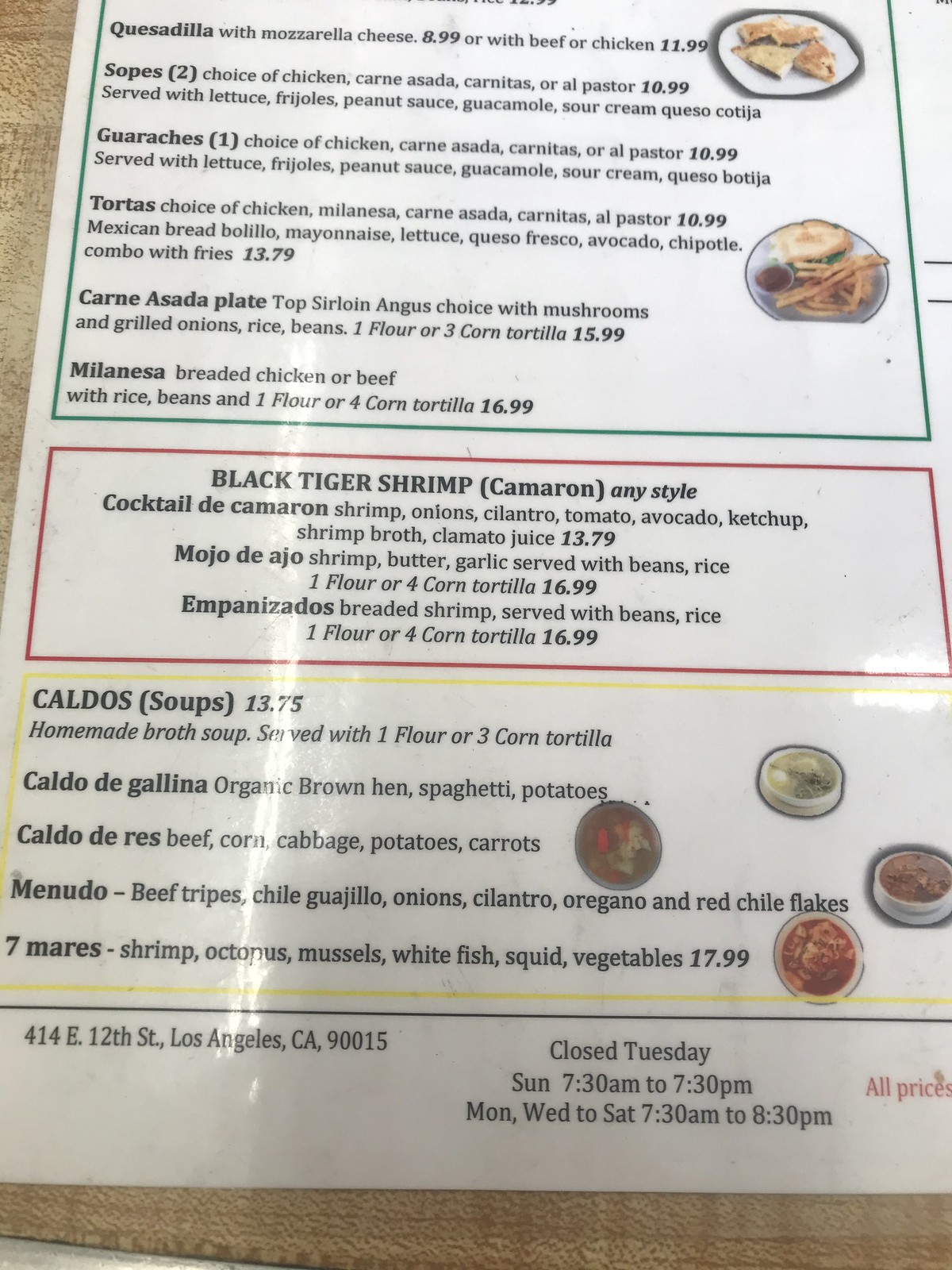The image features a detailed menu, displaying a variety of dishes and their prices. At the top, the menu lists options with mozzarella cheese priced at $8.99, and choices with beef or chicken for $11.99. Below those options, there is a section titled "Sopes."

Adjacent to this section, there is a bar or container with what appears to be bread. The next item on the menu highlights a "Top Sirloin" meal, which includes a garnish on the plate. It is listed with ingredients such as mushrooms, onions, rice, beans, one flour tortilla, and three corn tortillas, priced at $15.99.

Following this is another meal option: breaded chicken and beef, served with rice, beans, one flour tortilla, and four corn tortillas, priced at $2.69.

Further down, a red rectangle contains details about "Black Tiger Shrimp" served with French cheese and camaroni in any style, including cocktail form with shrimp and onions.

At the bottom of the menu, a yellow rectangle outlines a selection of soups made with homemade broths. These soups come with one flour tortilla and three corn tortillas, and feature organic brown heads, beef, corn, potatoes, carrots, beef, onions, cilantro, oregano, shrimp, octopus, mussels, and vegetables, priced at $17.99.

Additional information at the bottom left provides the address: 414 East 12th Street, Los Angeles, California, 90015, and indicates that the establishment is closed on Tuesday, Sunday, and Saturday.